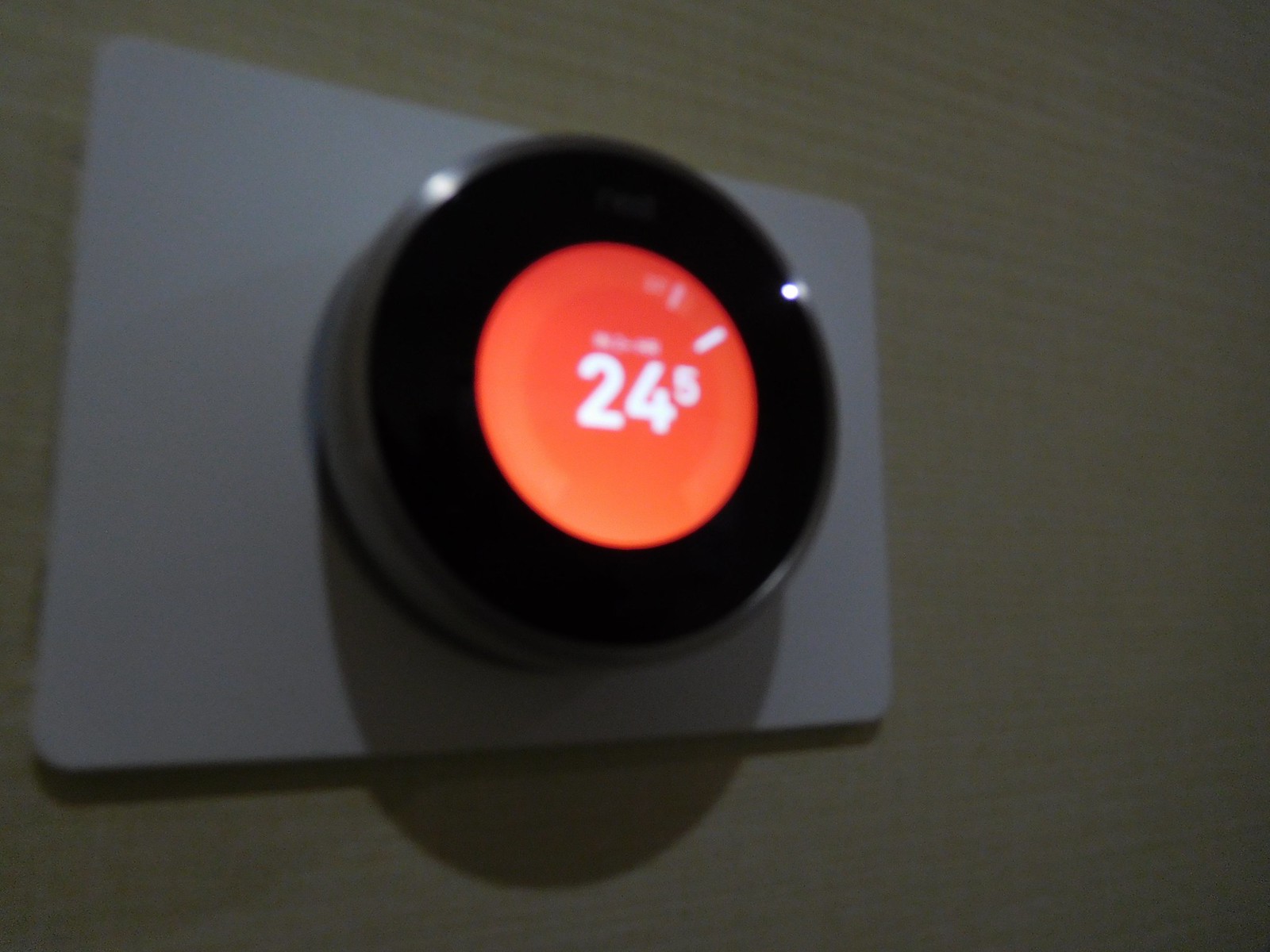A digital Nest thermostat is mounted on a textured, light yellowish-beige wall, which appears slightly out of focus. The wall itself features subtle horizontal lines, hinting at its texture. The thermostat is housed in a white plastic rectangle, with a circular, silvery center that includes a glass screen. Dominating the screen is a prominent red circle containing a white numeral '24.5', indicating the current temperature in degrees. Above this number, a small white line serves as an additional temperature marker. The photograph is taken in low light, casting a shadow from the device and contributing to the overall dark and shadowed appearance.